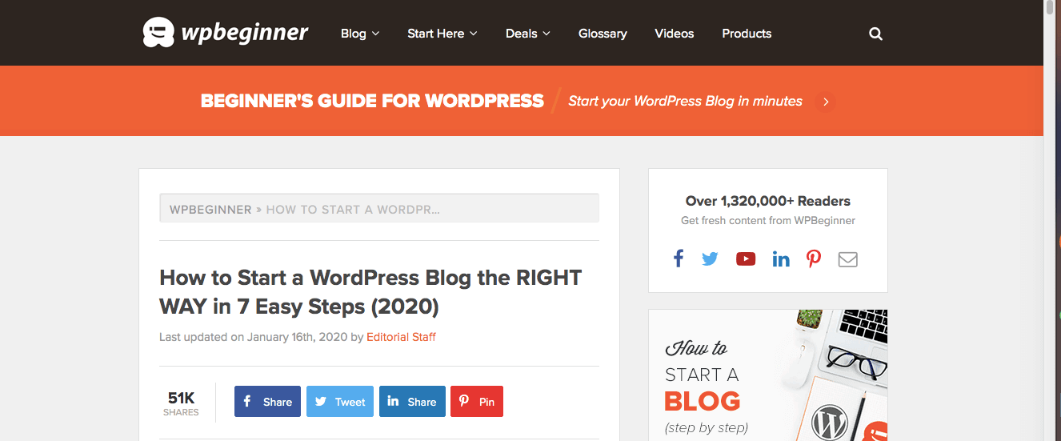**Detailed Caption:**

The image is a screenshot displayed in landscape mode. At the top section, from the upper left to the upper right, there is a brown stripe featuring the logo for WP Beginner. Adjacent to it are the tab headings: "Blog," "Start Here," and "Deals," each accompanied by a down arrow, followed by "Glossary," "Videos," "Products," and a search button.

Beneath this stripe lies a row with an orange background, bearing the text "Beginner's Guide for WordPress" prominently. Below that, in italics, the phrase "Start your WordPress blog in minutes" is followed by a right arrow icon.

In the main content area, the background is gray. To the right, there is a section with a white background containing a search bar and the title "WP Beginner: How to Start a WordPress." Below the title, it states "How to Start a WordPress Blog the Right Way in 7 Easy Steps," with a note that it was last updated on January 16, 2020, by the editorial staff. The "editorial staff" text is a live link. Additionally, the post has been shared 51,000 times and includes social media icons for sharing on Facebook, Twitter, LinkedIn, and Pinterest.

On the right side of this section, there is a highlighted message indicating that over 1,320,000 readers get content from WP Beginner. Below this, there is a heading that reads "How to Start a Blog Step-by-Step."